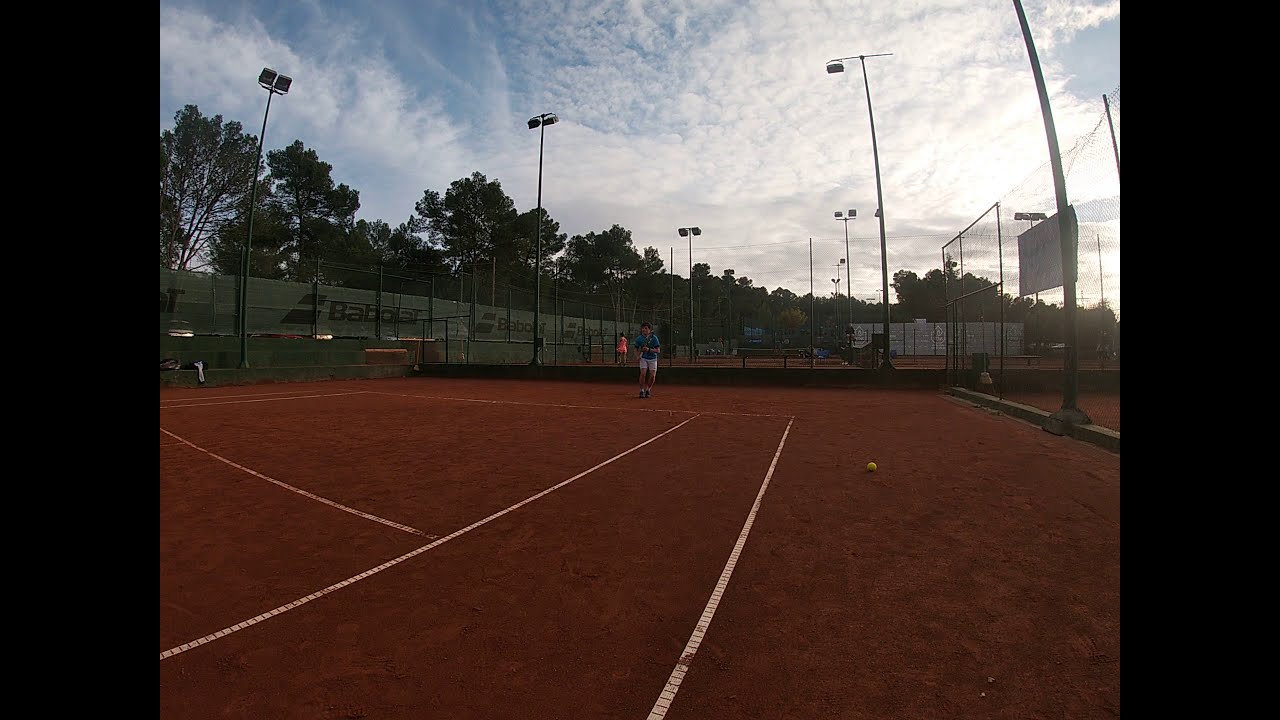The image captures an outdoor tennis court at a park, characterized by its brown clay surface and white painted lines. The court is framed by a fence on the right and a wooden wall on the left. Positioned directly in the center of the image is a person wearing white shorts and a blue shirt, standing behind the end line. The photo suffers from poor lighting due to low sunlight that is partially blocked by a sign on the right side. The sky above features white clouds. Surrounding the court are several light poles, though the lights are not turned on. Additionally, a ball, possibly a softball or baseball, is visible on the ground near the court.